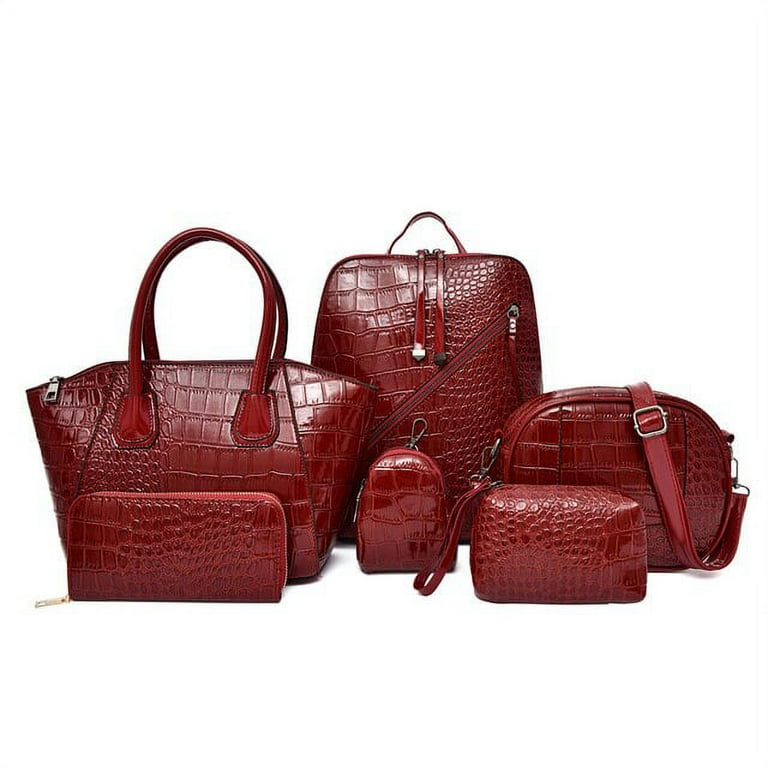This image showcases a collection of upscale handbags and purses, all crafted with a sophisticated animal skin texture, resembling alligator or snake skin patterns. Unified in a deep maroon or blood-red color, the variety includes different shapes and sizes, each designed for a unique purpose. At the center, a large handbag with red handles and a prominent silver zipper stands out. To its left, a large crossbody bag is accompanied by a matching small rectangular wallet with a similar texture design. Dominating the bottom center is a very small U-shaped bag with a zipper running over the top. On the right, there's a round or oval-shaped handbag, characterized by a long strap with metal buckles, paired with an adjacent compact makeup bag, almost square in shape. The high-quality, textured leather of these purses, set against a stark white background, highlights their rich color and intricate designs, making them visually striking and evidently designed for a discerning female clientele.